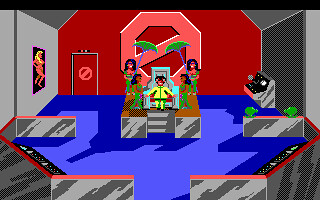The image appears to be a screenshot from a classic video game, characterized by its crude pixelated graphics. The setting seems to be a room with grey walls and a dark red back wall, featuring a lighter red octagonal shape bisected by a line. At the center of this room is a grayish-silver throne with a person seated on it, wearing a yellow shirt and green pants. Flanking the throne are four women, two on each side. The floor is adorned with a blue carpet or rug. Hanging on the wall behind the throne is a picture of a woman. There's also a doorway visible on the back wall and some sort of machine situated against the right wall.